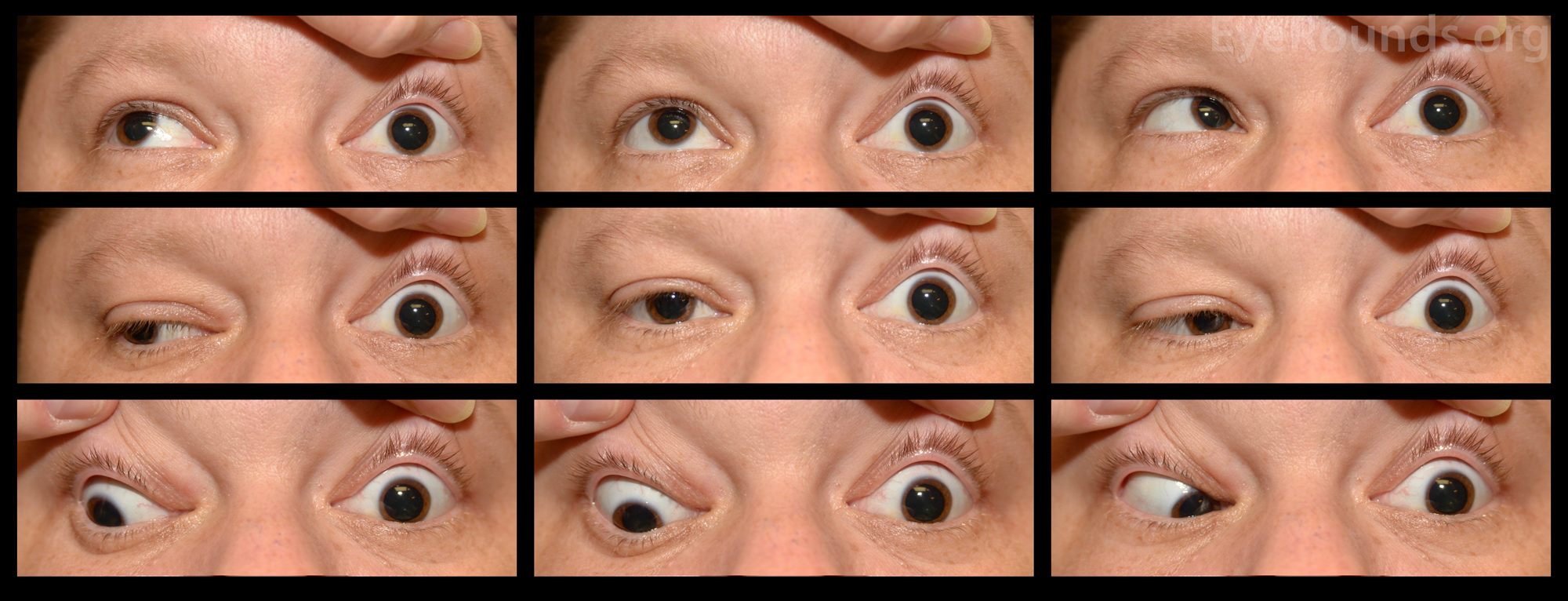The image features a 3x3 grid of close-up photographs focusing on a person's eyes, likely from an eye exam. Each of the nine photos captures both eyes of a light-skinned individual with light-colored eyebrows, brown eyelashes, and light brown irises. The photographs, taken from just above the nose to the lower forehead, display the eyes looking in various directions: left, right, center, and downward. A prominent detail across all images is the presence of a hand, frequently holding up the skin around the eyes to widen the eyelids, possibly for medical assessment. The person’s right eye (viewer’s left) appears narrower in multiple images, perhaps suggesting an eye condition. The sequence in the grid correlates the direction of the eyes to their position in the grid; for example, the eyes look towards the top-left in the top-left photo, and towards the bottom-right in the bottom-right photo. The watermark “irounds.org” in the top-right corner of the grid suggests the images are from an eye health organization.